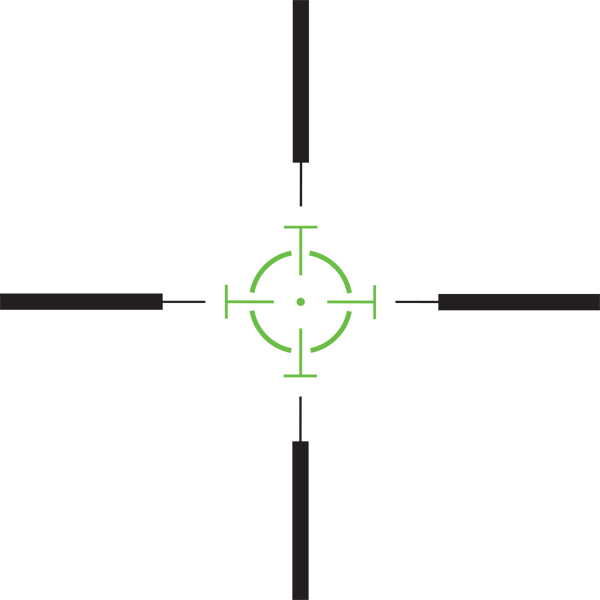The image is a detailed graphical depiction of a crosshair resembling a target. It features a white background and consists of several distinct components. At its core is a green circle with a green dot at the center. Extending outward from this central circle are four green arms, each terminating in perpendicular bars, forming a shape reminiscent of capital T's pointing in the north, south, east, and west directions. Encircling this are four black lines, each connected to the circle's outer perimeter. These black lines are thin and stretch outwards, ending in longer black rectangles, positioned at the top, bottom, left, and right. The overall design is clean, synthetic, and devoid of any text, focusing purely on the geometric alignment and contrast of colors and shapes, which together resemble a precise target or crosshair mechanism.